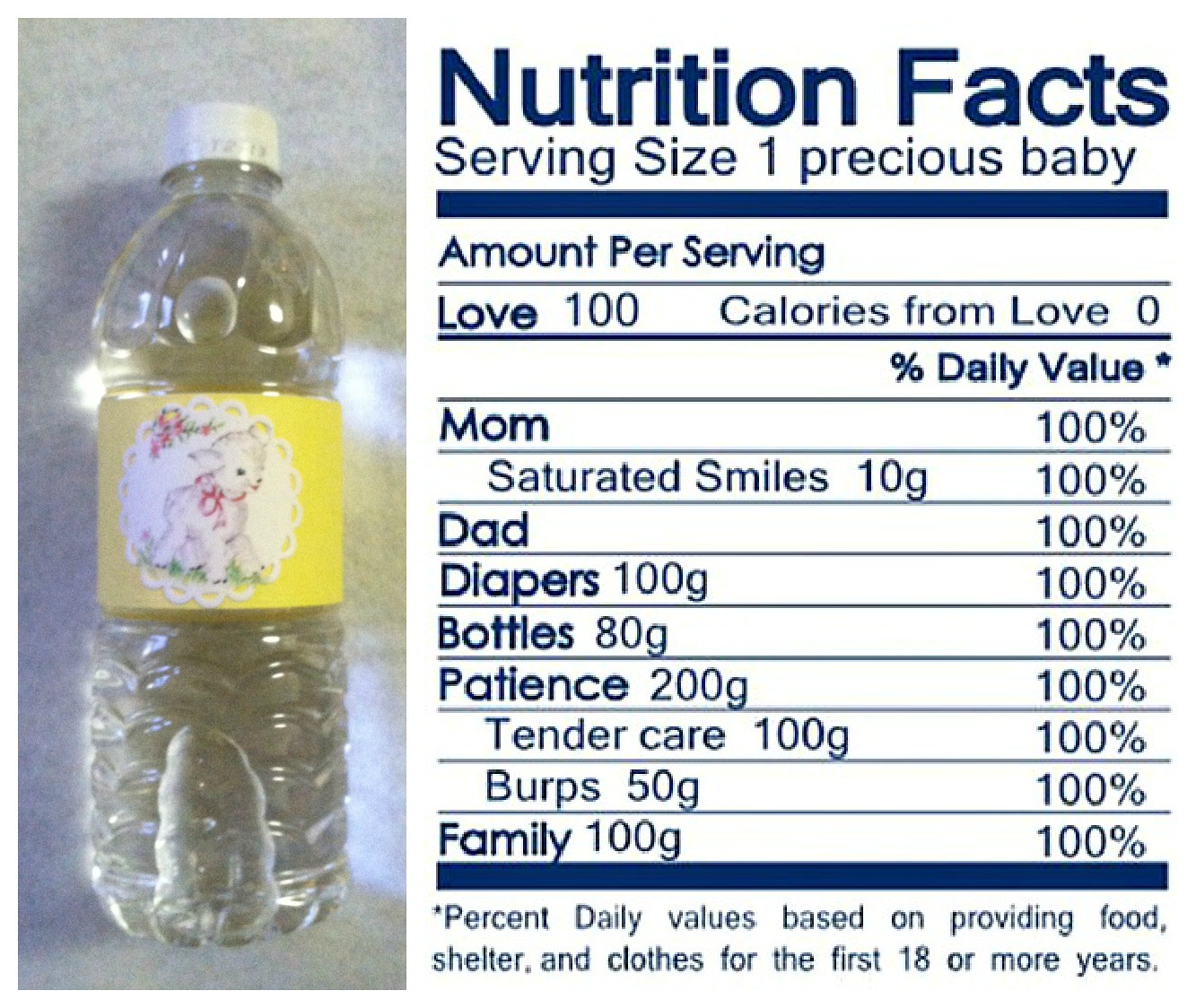The photograph features a clear plastic bottle filled with liquid, capped with a white lid, resting on a mottled gray surface. The light source is positioned on the left side, creating reflections on the right side of the bottle. The bottle's label is a cheerful, sunshine-yellow color. Prominently displayed on the label is an oval-shaped white image depicting a lamb with a red bow around its neck, standing on grass and facing right.

The nutrition facts on the label add a whimsical touch: 
- Serving Size: One Precious Baby
- Amount Per Serving: Love 100 calories, Calories from Love 0

The percentage daily values are creatively listed:
- Mom: Saturated Smiles 10 grams, 100%
- Dad: 100%
- Diapers: 100 grams, 100%
- Bottles: 80 grams, 100%
- Patience: 200 grams, 100%
- Tender Care: 100 grams, 100%
- Burps: 50 grams, 100%
- Family: 100 grams, 100%

An additional note humorously indicates that the percent daily values are based on providing food, shelter, and clothes for the first 18 or more years.